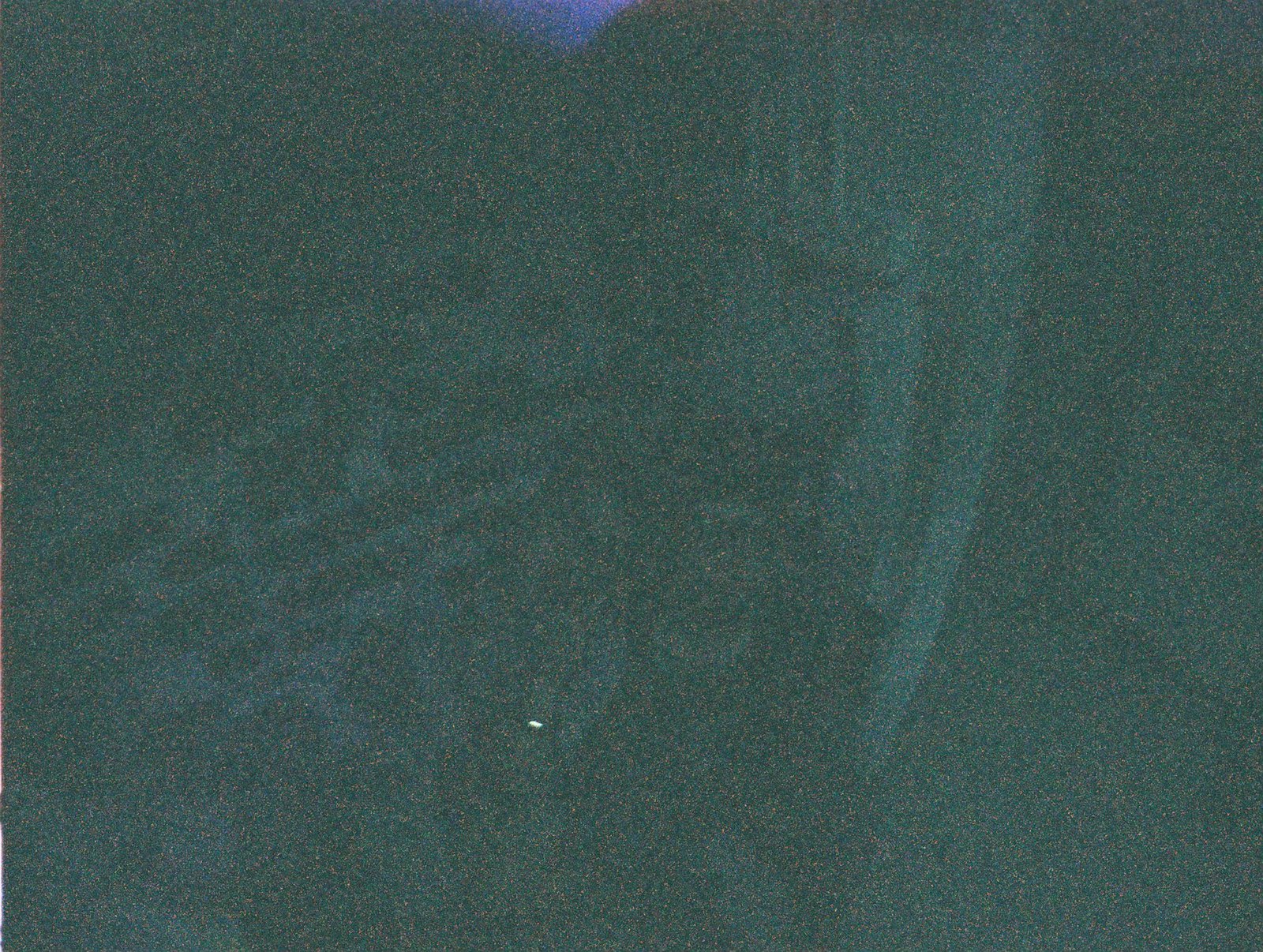This horizontal landscape-oriented image captures an outdoor scene, though its precise subject is difficult to discern due to the dark and grainy quality. The overall dominant color is a dark pine green, reminiscent of a blanket or fabric. Light plays across the surface, creating a series of lighter green lines and rub marks, particularly noticeable on the right side with vertical alignments and on the barely visible left side with horizontal ones. A hint of blue at the top center of the image adds subtle contrast. There is also a small white line about three inches from the bottom, suggesting the top edge of an object, possibly a blanket. The texture appears smooth, akin to suede or similar material, and tiny particles of yellow and green can be seen interwoven within the fabric.